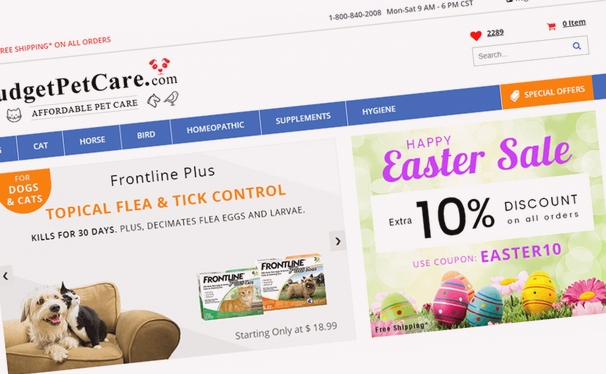The webpage appears slightly tilted, but prominently displays "REE" in red at the top, suggesting the full name might be "FREE" though the 'F' is cut off. To the right, a black text provides a contact number: "1-800-840-2008." Below this, operating hours are listed as "MON-SAT 9AM-6PM CST." A thin gray line separates this information from the partially visible black text "D-G-E-T-Petcare.com."

Above this text, there's an icon resembling a poop emoji. Beneath, a black-and-white cat is pictured on the left side, and on the right, a horse head and a bird are depicted. Between these images, the phrase "Affordable Pet Care" is written in black, bracketed by gray lines above and below. Nearby, a red heart is shown with the number "2289" underlined in black next to it.

A red cart icon indicates "zero items" underlined. Below, a white search box outlined in gray is labeled with "Search," in capital 'S' gray text, followed by ellipses "..." and a blue magnifying glass icon on the left side. 

The blue-bordered section beneath lists categories: "cat, horse, bird, homeopathic supplements, hygiene," followed by an orange rectangle offering "special offers." Detailed in white text, it includes "Front Line Plus Topical Flea and Tick Control – kills for 30 days, decimates flea eggs and larvae, starting at $18.99." The announcement "Happy Easter Sale" is highlighted in purple with a black note: "Extra 10% off discount on all orders."

Overall, the page integrates essential contact information, service hours, product offerings, promotional details, and navigational elements for an online pet care store.